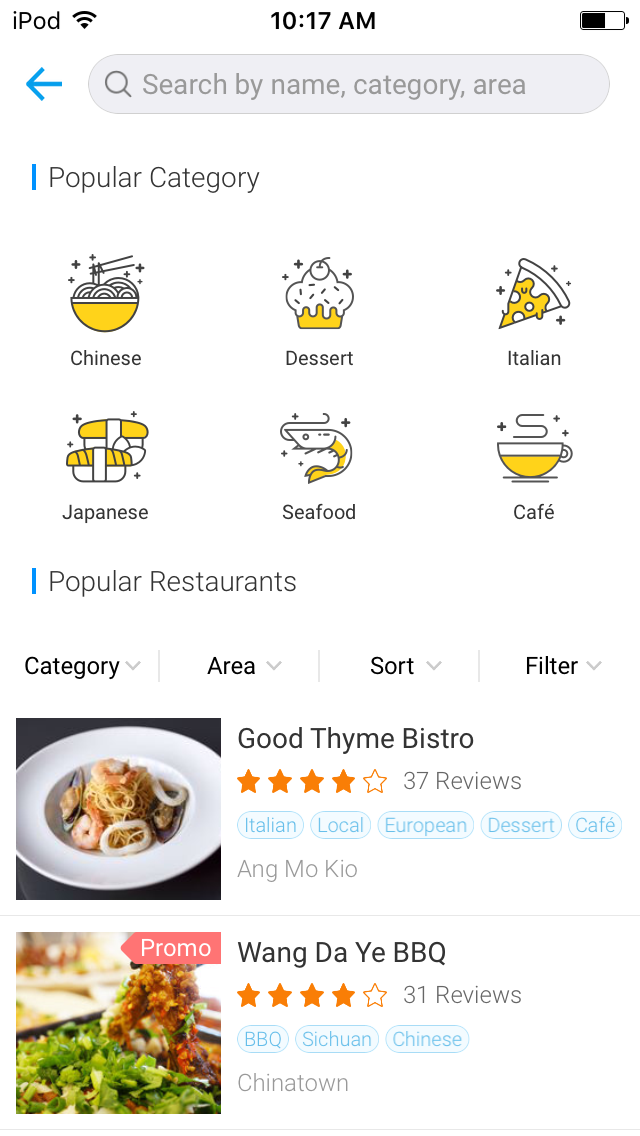This is a screenshot from a cell phone displaying a popular category section for restaurant choices. The interface showcases a search area for restaurants, highlighting six popular categories organized in two rows of three. The top row features "Chinese," "Dessert," and "Italian," while the bottom row includes "Japanese," "Seafood," and "Cafe." Each category is visually represented by an intuitive icon: a cupcake for "Dessert," a pizza slice for "Italian," a fish for "Seafood," and a teacup for "Cafe." Below these categories is a section for popular restaurants, where the first listing shows "Good Thyme Bistro," which cleverly uses the herb "thyme" in its name. The restaurant boasts a rating of four stars based on 37 reviews.